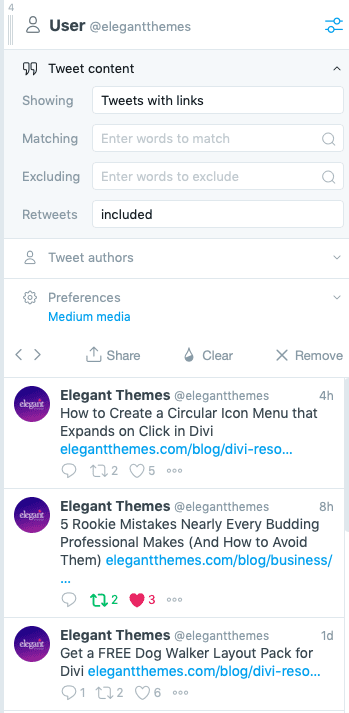The image appears to be a screenshot from a mobile phone, displaying a Twitter search interface. In the upper left corner, there's an icon resembling a stylized person, indicating the user is associated with "Elegant Themes." 

Beneath this, the text "tweet content" is enclosed in quotation marks, suggesting a search or filtering criterion for tweets. Following this, "showing" is mentioned, accompanied by a rectangle labeled "tweets with links," indicating a filtered view of tweets containing links. Directly below this, the word "matching" appears next to a search box labeled "enter words to match."

Adjacent to this section is the word "excluding," with a corresponding search box labeled "enter words to exclude." Below this, the text "retweets" is displayed, with a box on the right showing the word "included," suggesting that retweets are part of the search criteria. The phrase "tweet authors" is listed next, followed by "preferences."

Further down, the terms "media" and "media" appear, likely indicating additional filtering options. At the bottom of the screenshot, three posts are visible, each marked by the purple logo of Elegant Themes. 

- The first post reads: "How to create a circular icon menu that expands on click in DIV."
- The second post states: "Five rookie mistakes nearly every betting professional makes (and how to avoid them)."
- The third post promotes: "Get a free dog walker layout pack for Divi."

This detailed capture highlights the use of the Elegant Themes interface for refining and browsing specific types of tweets.